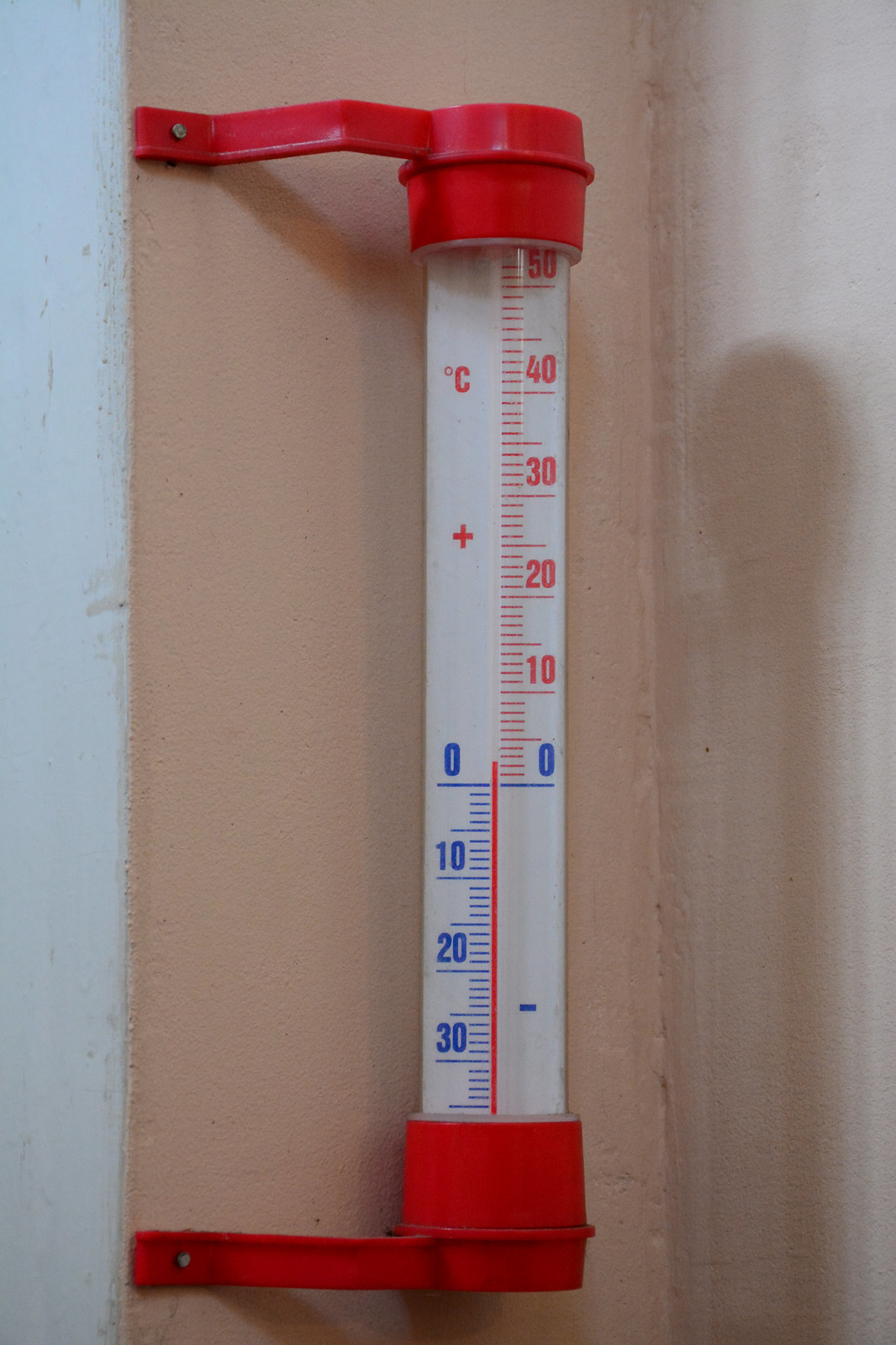The image is a vertical photograph of an outdoor thermometer, which is securely mounted on a rose-colored wall. The wall features a white border running vertically along the left side of the image, adding a distinct contrast to the warm background. The thermometer is affixed to the wall with two red-painted metal strips bent into brackets that hold it firmly in place. Each bracket is attached using a small-headed nail or brad driven through a hole in the metal strip.

The thermometer itself is encased in a clear cylindrical tube, which could be made of glass or plastic. The internal scale of the thermometer displays temperatures in degrees centigrade, clearly marked for easy reading. The upper two-thirds of the scale represent the positive temperature range, marked in red, and span from 0 to 50 degrees Celsius with horizontal graduation lines for precision. The lower third of the scale indicates the negative temperature range, marked in blue, and spans from 0 to -35 degrees Celsius. The neat, incremental markings and vivid color differentiation between the positive and negative ranges make this a practical and visually appealing outdoor thermometer.